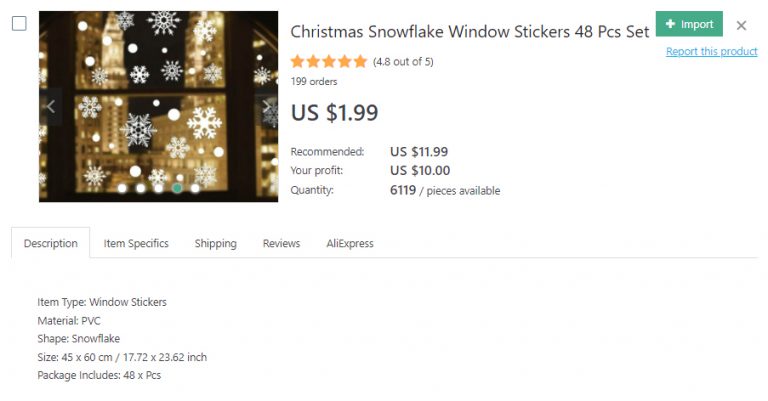This detailed caption describes the screenshot:

"The screenshot is from an online storefront showcasing a product listing for 'Christmas Snowflake Window Stickers.' The featured item is a set of 48 PVC snowflake-shaped stickers designed for window decoration. The stickers are displayed adhered to a glass door pane, creating a festive winter scene with various sizes of intricate snowflakes interspersed with small dots resembling additional snow. The product has received a high rating of 4.8 out of 5 stars based on 199 orders, priced at $1.99 USD after discount from the recommended $11.99, allowing for a $10 profit margin. There is substantial stock available, with 6,119 pieces in inventory. The listing provides an item description, specifying the material as PVC and the size as 45 by 60 centimeters (17.72 by 23.62 inches), with the package containing 48 pieces. Additional tabs on the product page offer detailed item specifics, shipping information, customer reviews, and a link to the storefront on AliExpress."